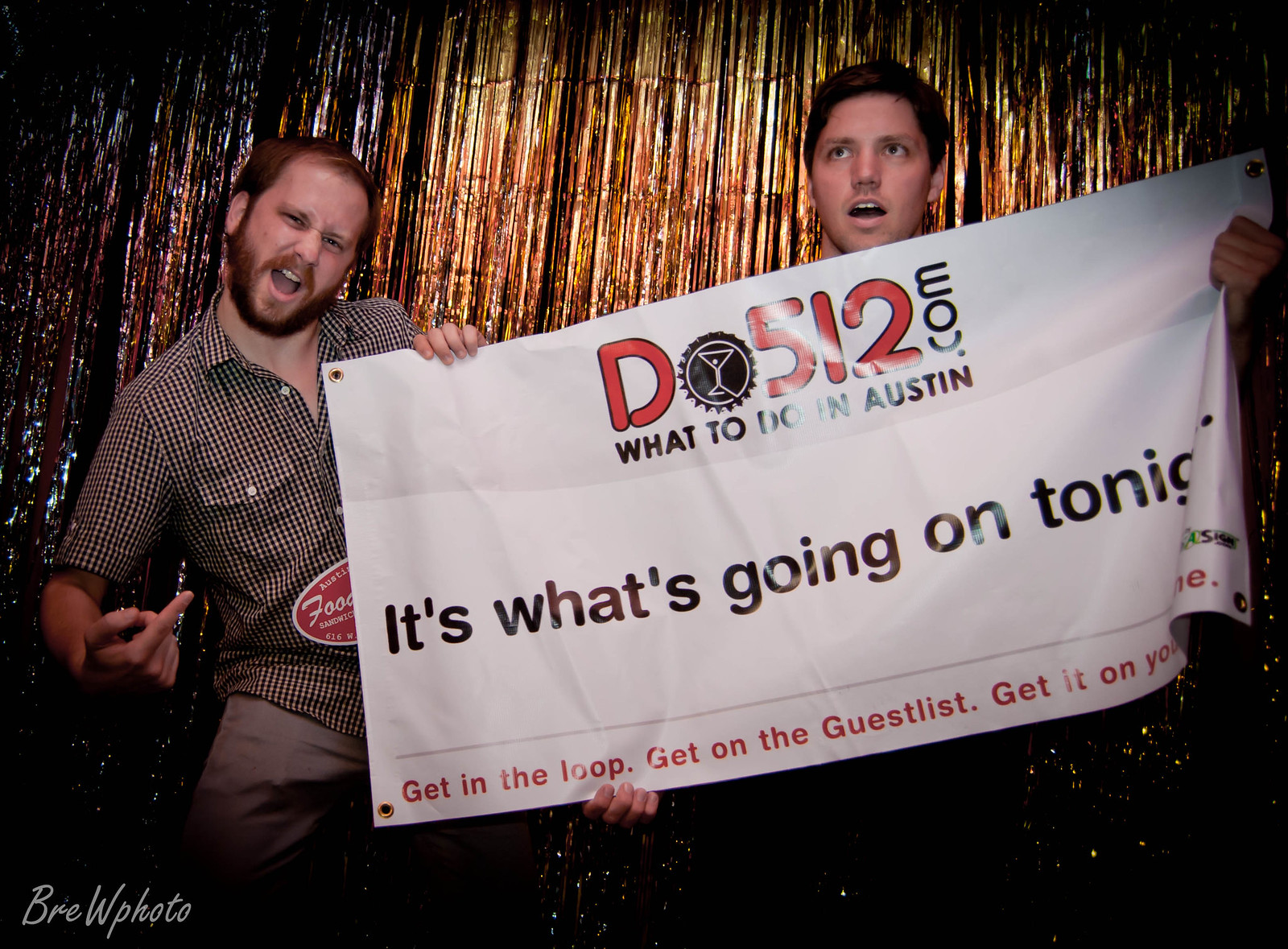In the image, two men stand in front of a metallic, gold-fringed curtain, holding a white sign with black and red text. The man on the left, with auburn hair, a mustache, and a beard, is wearing an open dark brown or black checkered shirt and khaki pants. He is pointing to the sign with his right hand, mouth open in a "hey" expression, and squinting slightly, his left hand adorned with several rings. The man on the right, only visible from the neck up, holds the sign in both hands and gazes upwards with an open mouth. The white sign they are holding is divided into three sections. 

The top section features red text and a black bottle cap and martini glass graphic, reading "DO512.com," followed by "what to do in Austin." The middle section, on a white background, states "what's going on tonight." The bottom section has partially cut-off red text, "get in the loop. Get on the guest list. Get it on your," with the last word obscured due to the poster's fold. The lower left corner of the sign bears the watermark "Brie W photo," presumably the photographer's credit. This photograph, likely an advertisement, highlights an event guide for Austin, Texas.